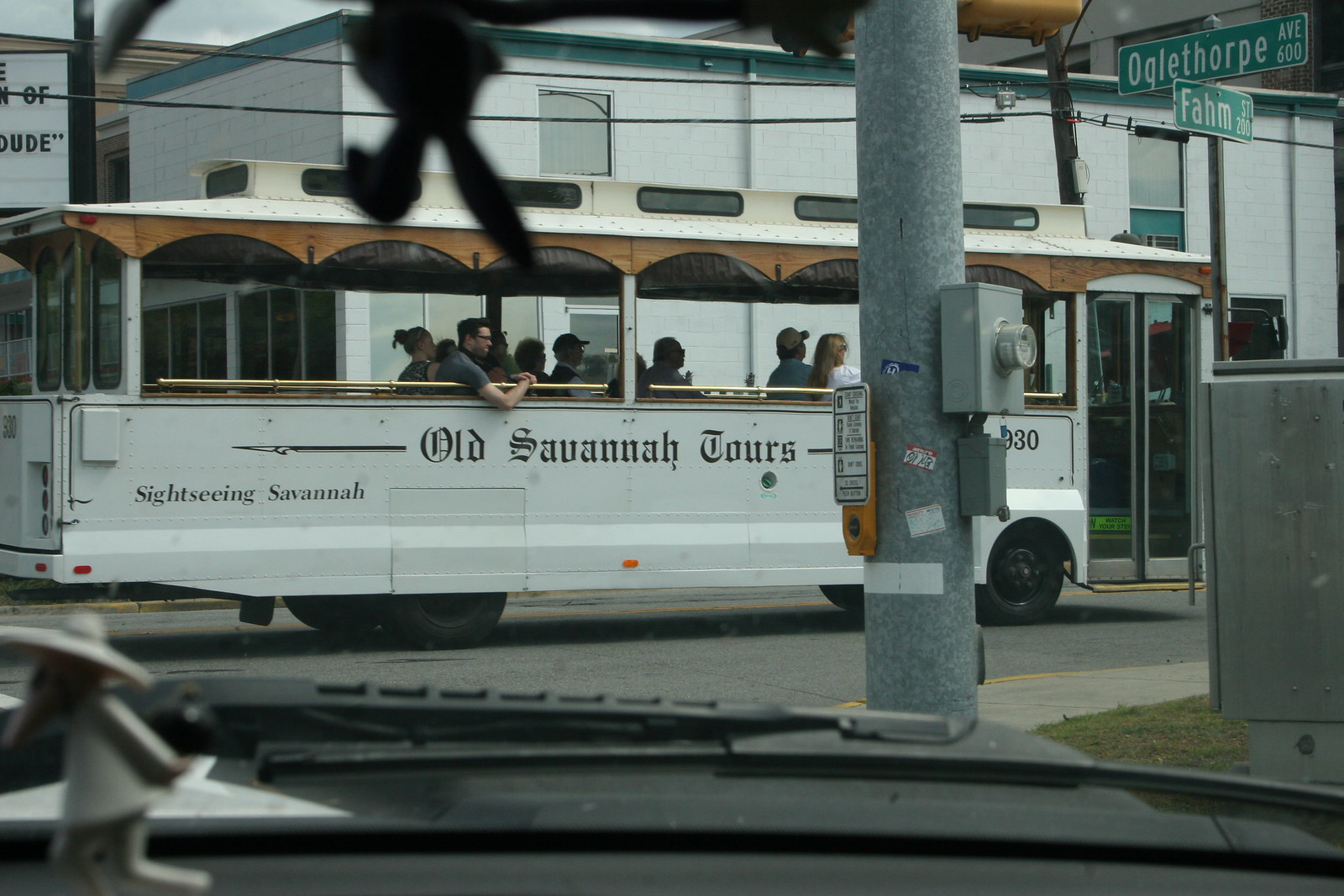The photograph depicts an urban scene taken from the dashboard of a car waiting at the intersection of Oglethorpe Avenue and Fahm Street (600 block of Oglethorpe Avenue and the 200 block of Fahm Street) in downtown Savannah, Georgia. The image, slightly dark due to possible tinted windshield exposure, shows a white, open-window tour bus, 'Old Savannah Tours', with brown curtains around the roof's edges and "Sightseeing Savannah" written on its side in Old English font. The bus, with about a dozen passengers, appears to be an open carriage, with some individuals hanging out of the windows enjoying their tour. To the right of the image, there's a concrete wall, and above it, a street sign indicating the intersection. A lamppost with a pedestrian crossing button is visible, and further behind, a one-to-two-story commercial building can be seen, enhancing the urban atmosphere of this historic city.